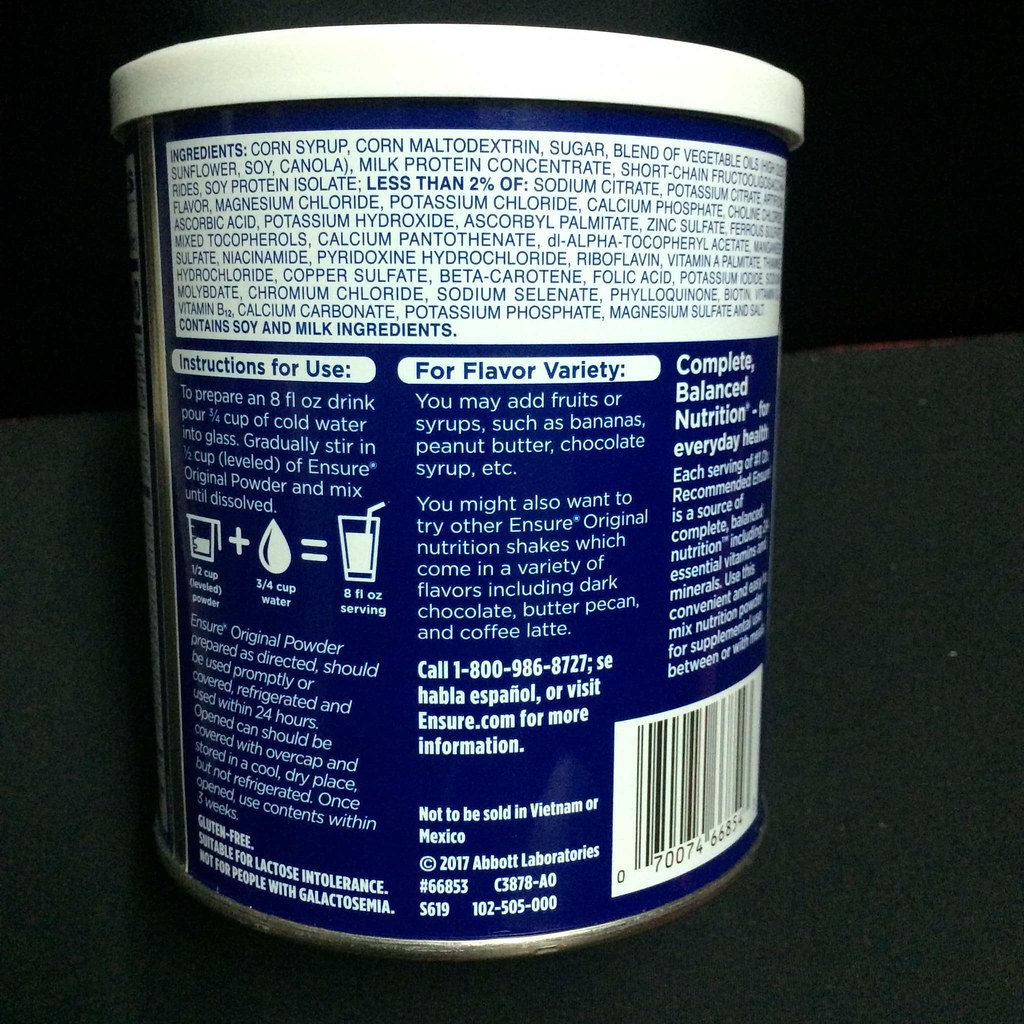This image is a close-up photograph of the back of a canister that appears to be a container of Ensure. The canister has a white plastic lid atop a predominantly blue base with a metal bottom. A white label covers the upper part of the can, listing a long array of ingredients in blue text. Below this, a banner outlines detailed instructions for preparing an 8-ounce drink: pour one-quarter cup of cold water into a glass, then gradually stir in one half cup of Ensure Original powder until dissolved. The instructions are also visually represented with a diagram that includes a glass, a drop of water indicating 3/4 cup, and a glass nearly filled to 8 fluid ounces with a straw. The bottom right corner prominently displays a barcode, accompanied by a note indicating the product should not be sold in Vietnam or Mexico, and includes a copyright notice from Abbott Laboratories, dated 2017. Additional suggestions are provided for flavor variety, recommending the inclusion of fruits or syrups such as bananas, peanut butter, or chocolate syrup. The label also features a 1-800 number and the address of Abbott Laboratories for customer service inquiries.